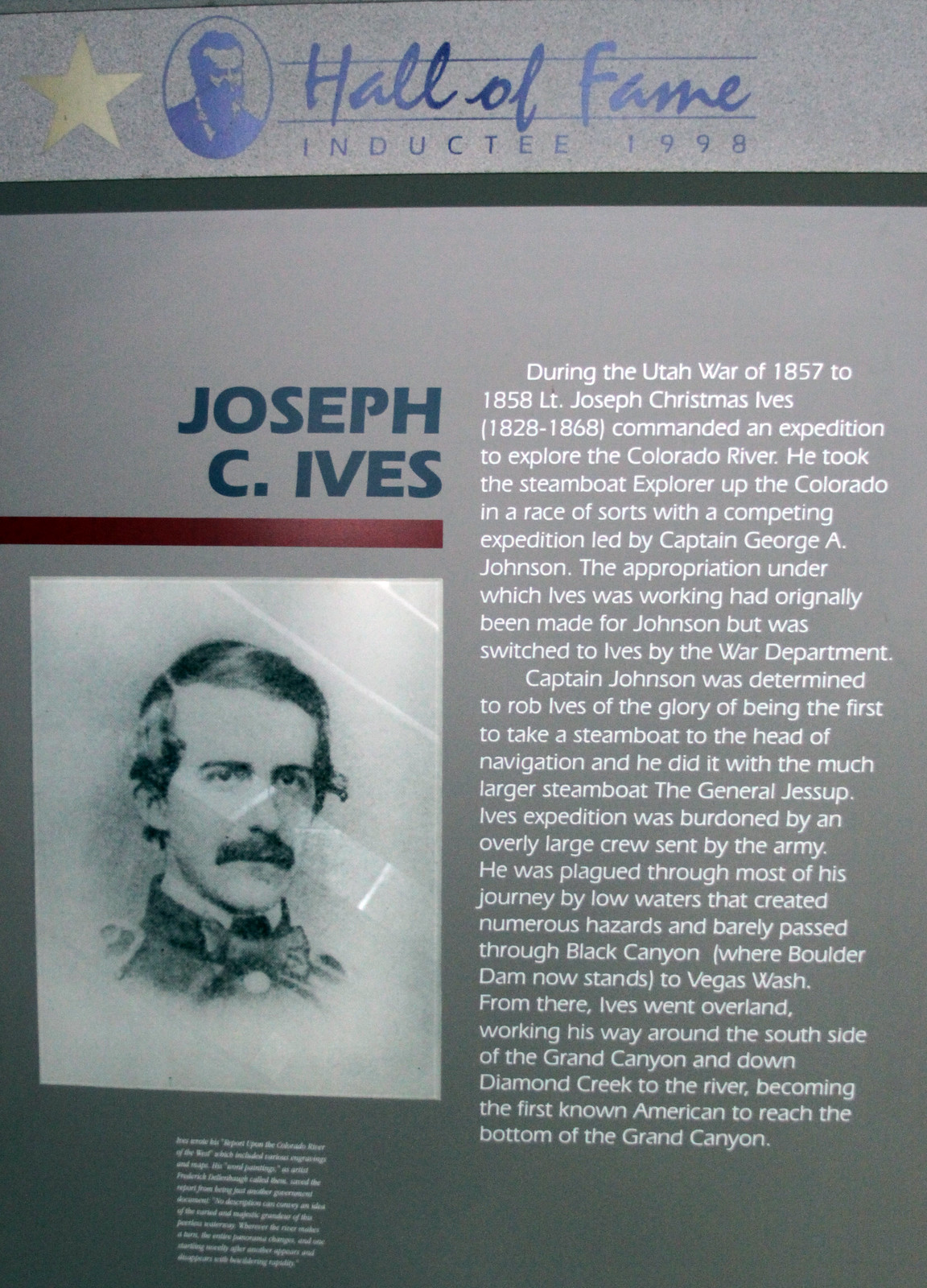This image depicts an exhibit with a gray background and blue accents, resembling a museum plaque. At the top, within a blue circle, is a drawing of a bearded man accompanied by blue cursive text that reads "Hall of Fame." Below, it declares "Inductee 1998." Centered in the exhibit is an old black-and-white photograph of a white man with a mustache and slicked, slightly curly black hair, reminiscent of Civil War-era portraits. The man's name "Joseph C. Ives" is displayed prominently above the photo. To the right, a detailed account provides a historical narrative about Lieutenant Joseph Christmas Ives (1828-1868), emphasizing his role during the Utah War of 1857-1858. It recounts his command of an expedition to explore the Colorado River aboard the steamboat Explorer, amid a competitive race with Captain George A. Johnson. Despite facing challenges like an overly large crew and hazardous low waters, Ives navigated through Black Canyon, reaching Vegas Wash. He later traversed overland, circumventing the Grand Canyon to descend Diamond Creek, ultimately becoming the first known American to reach the bottom of the Grand Canyon.